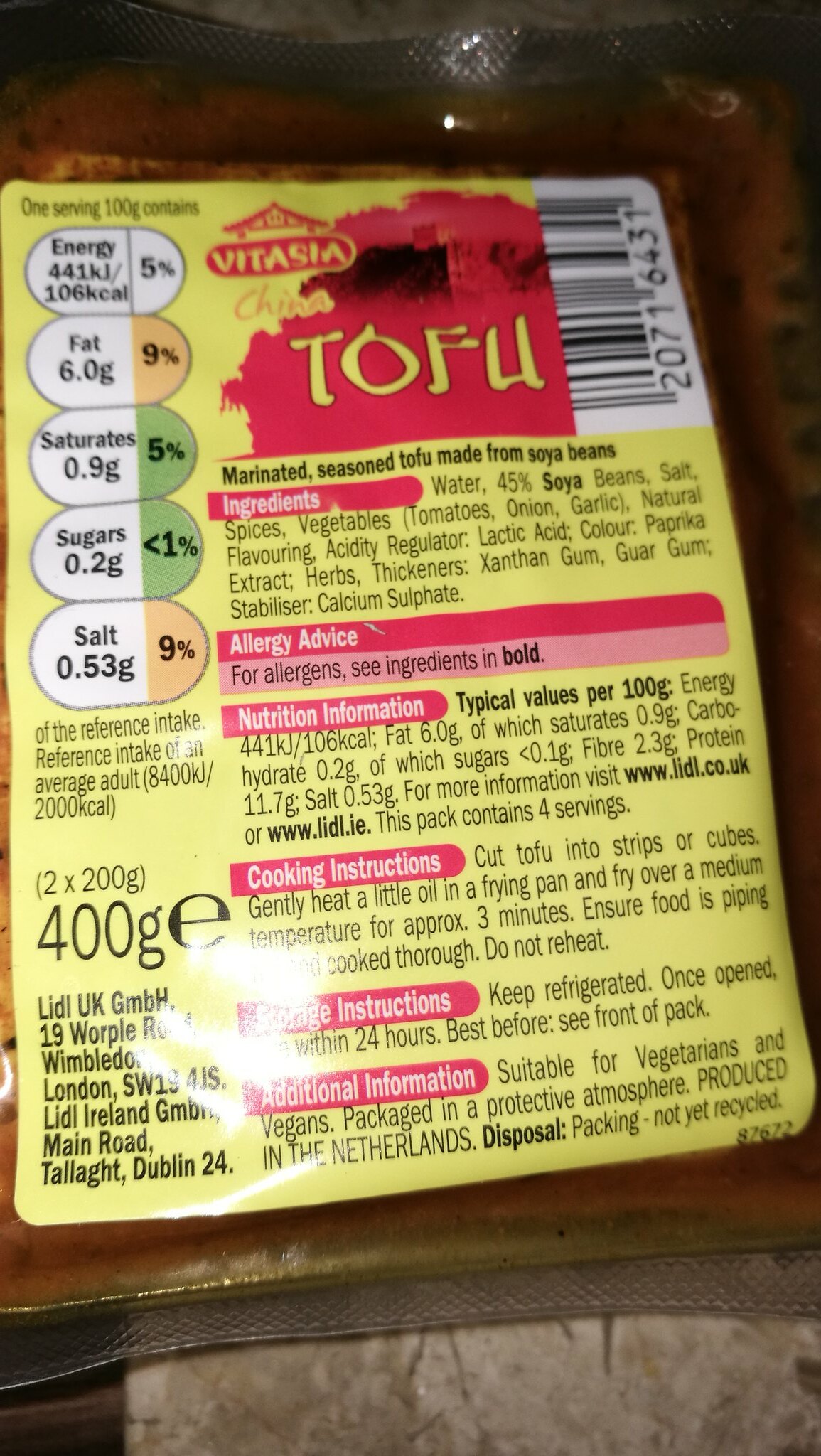Detailed Caption: 

The image showcases a brightly colored yellow pack of tofu. Prominently displayed on the front is the brand name "Vida Ziza," positioned above the product label "China Tofu." The packaging indicates a net weight of 100 grams. The front of the pack is densely populated with text, detailing nutritional benefits and information: it specifies 5% fat, 9% saturated fats, and 5% sugars. The packaging also includes a comprehensive breakdown of ingredients, allergy advice, and nutritional facts. Although partially obscured by glare, cooking and storage instructions are also provided. The overall design is informative, emphasizing clarity and consumer guidance.